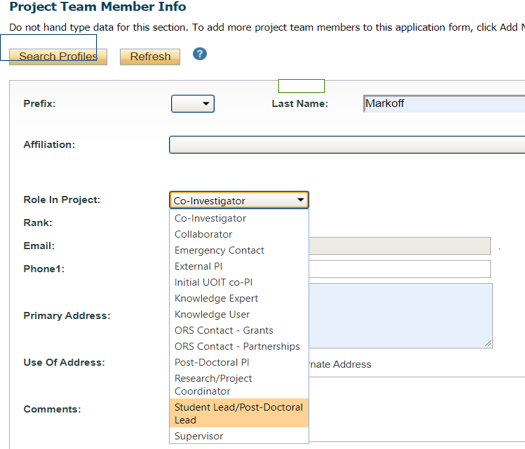In this image, a screenshot captures a detailed interface of an academic information portal designed for entering research project details. The interface features a clean white background contrasted with black text. Users are prompted to fill out several fields associated with their personal and professional information. These fields include prefix, last name, affiliation, role in the project, rank, cell phone number, primary address, use of address, and comments. 

A notable aspect of the screenshot is a drop-down menu, currently showcasing a selection of roles within the project. This menu includes multiple options such as Co-investigator, Collaborator, Emergency Contact, and more. The specific role highlighted in orange is "Student Lead/Post-doctoral Lead," indicating the individual filling out the form holds this position. 

Additional details reveal that the last name entered into the form is "Markoff" (spelled M-A-R-K-O-F-F). The layout is organized such that the labels for each field are positioned on the left, while the corresponding input areas for the information are aligned on the right. The ongoing nature of form completion suggests that this individual is in the midst of submitting their particulars for a research project, likely situated in the academic sector.